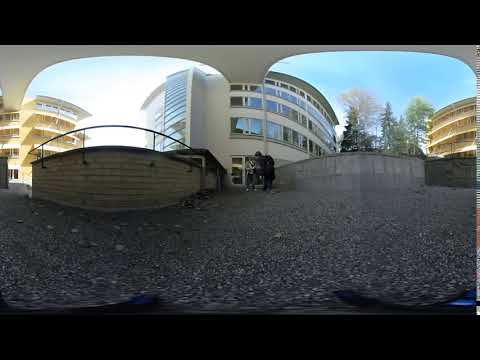The image features a striking building with a round architectural design, standing approximately four to five stories high. The building is adorned with numerous glass windows that encircle each floor, enhancing its modern aesthetic. The structure is primarily white, and one section includes balconies. Flanking the main building, though partially cut off by the camera, are two additional roundish buildings. 

In the foreground, a gravel area leads up to the structure, bordered by two rock walls on either side. A man dressed in black is seated on the wall to the right. In addition, the outdoor setting includes green trees, a blue sky, and scattered clouds, with a driveway visible as well. There are two people seen outside the building, although they appear blurry.

Interestingly, the image seems to exhibit some visual distortion, possibly due to VR 360 imaging. This warping effect makes the scene appear as if it could support activities like skateboarding or parkour, with railings and raised platforms visible on either side. The environment might be enclosed, suggested by what resembles a roof-like structure, adding to the unusual perspective.